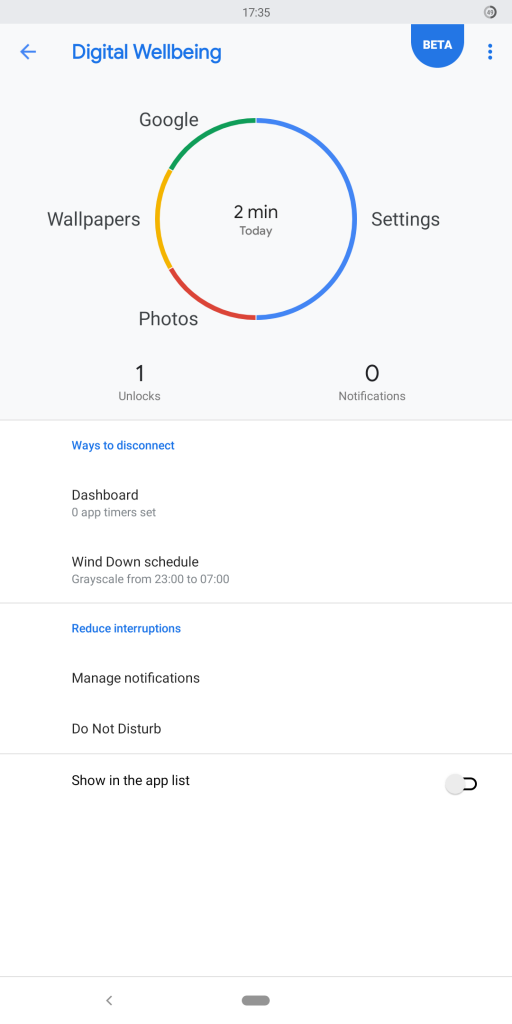The screenshot displays a 'Digital Well-being' dashboard with a sleek interface. At the top, a small gray band shows the current military time as 17:35. To the right, a small blue tab labeled 'BETA' indicates that the feature is in its testing phase.

Central to the image is the title 'Digital Well-being' in blue. Beneath the title, a multi-colored circle provides a visual breakdown of app usage: the green segment represents 'Google,' the yellow stands for 'Wallpapers,' the red for 'Photos,' and the blue for 'Settings.' Inside this usage circle, the text '2 minutes today' summarizes the total screen time for the day.

Below the circle, two lines of text display statistics: '1 unlock' and '0 notifications.' Further down the screen, several menu options are listed, including 'Dashboard,' 'Wind Down,' 'Schedule,' 'Manage Notifications,' 'Do Not Disturb,' and 'Show in the app list.'